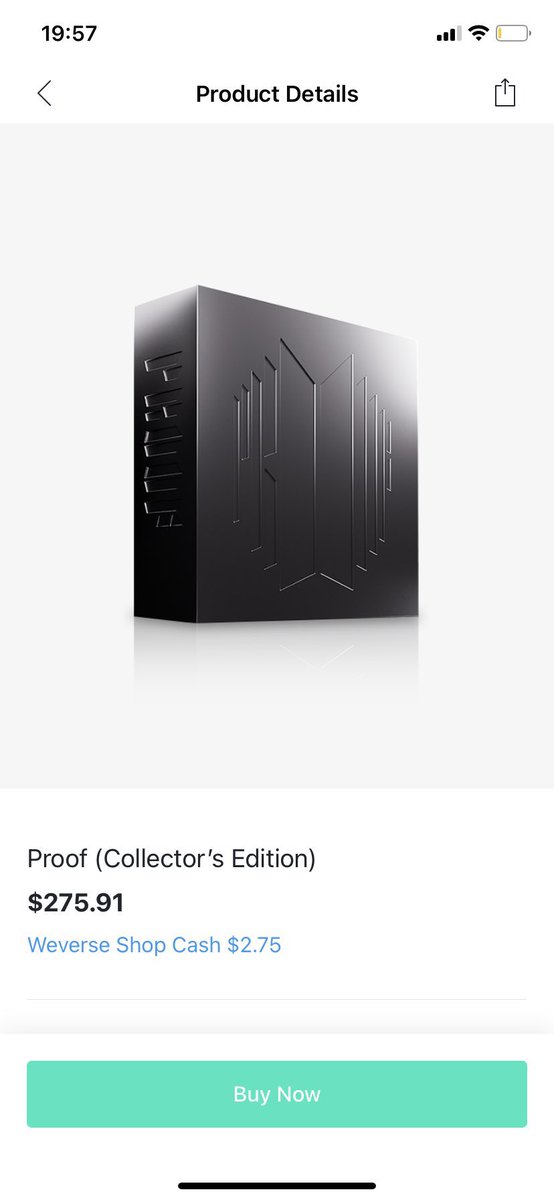The image displays a 1957 top flash indicator with three out of four bars, showing full Wi-Fi connectivity but an almost empty battery under battery-saver mode. Icons on the display include a left arrow, a right square, and an upward arrow. A central feature is a PC case, appearing as a black metal box with intricate etching. The shapes and edges are white, on a gray background. The bottom of the image has the text “proof (Collector's Edition)” priced at $75. Below this, "Weaver shop cash $2.75" is mentioned. A green rectangle in the middle contains the text “Buy Now.” At the bottom is a black bar with a subtle sheen from light at its center. The image's top left corner is white. The overall layout suggests it is viewed from a smartphone, as indicated by its rectangular form factor.